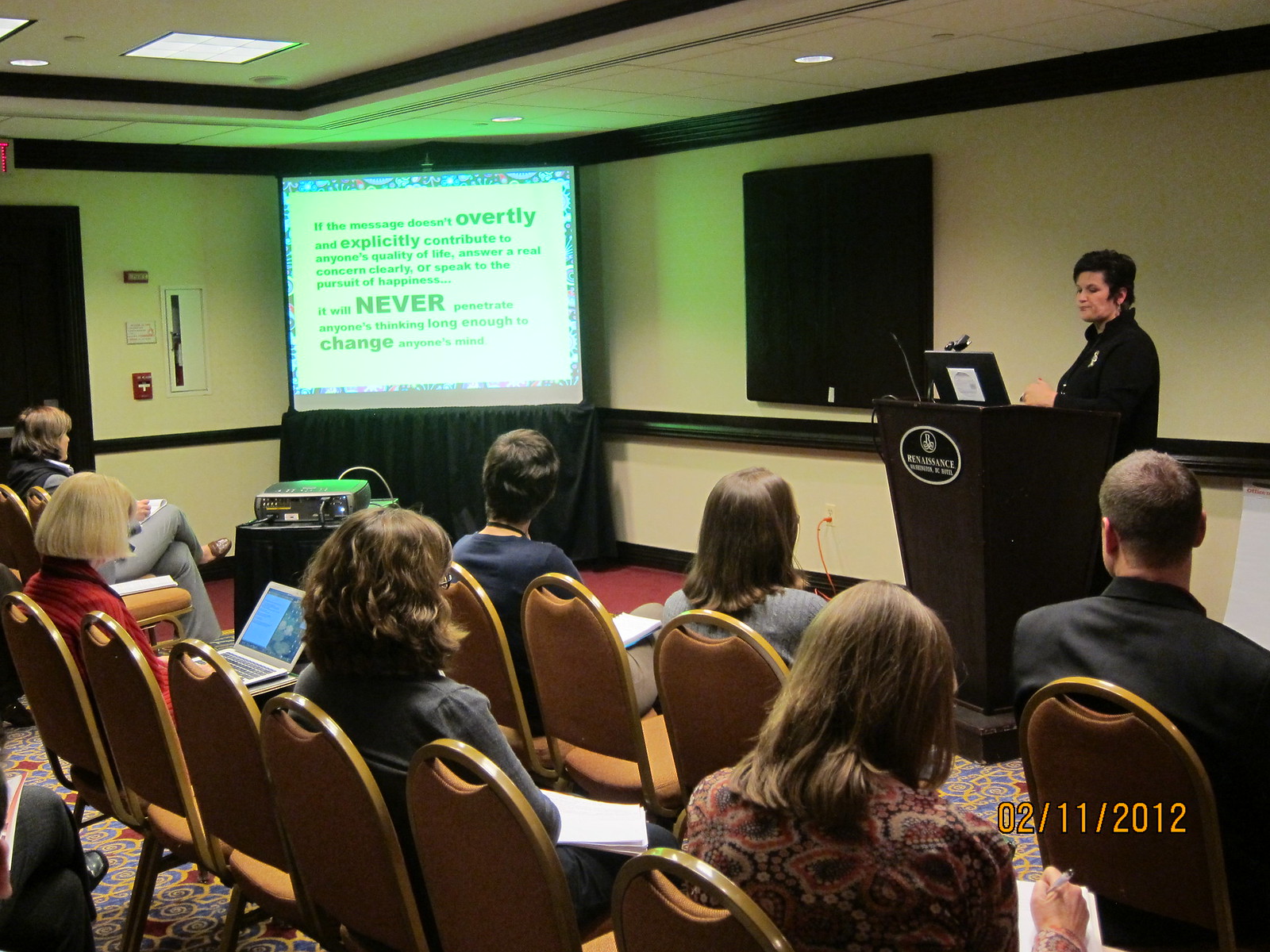In a warmly lit hotel conference room with neutral yellowish walls and black trim, a middle-aged woman with short black hair stands at a dark brown podium, giving a presentation. The podium holds a laptop, which she references as she speaks to an audience of about 15 people, seated on conference chairs facing her. The room features red carpeting with ornate floral designs and a projected screen to her right, displaying clipart and words in big green font. The audience, composed of both men and women, watches her intently, many taking notes as she delivers her talk.